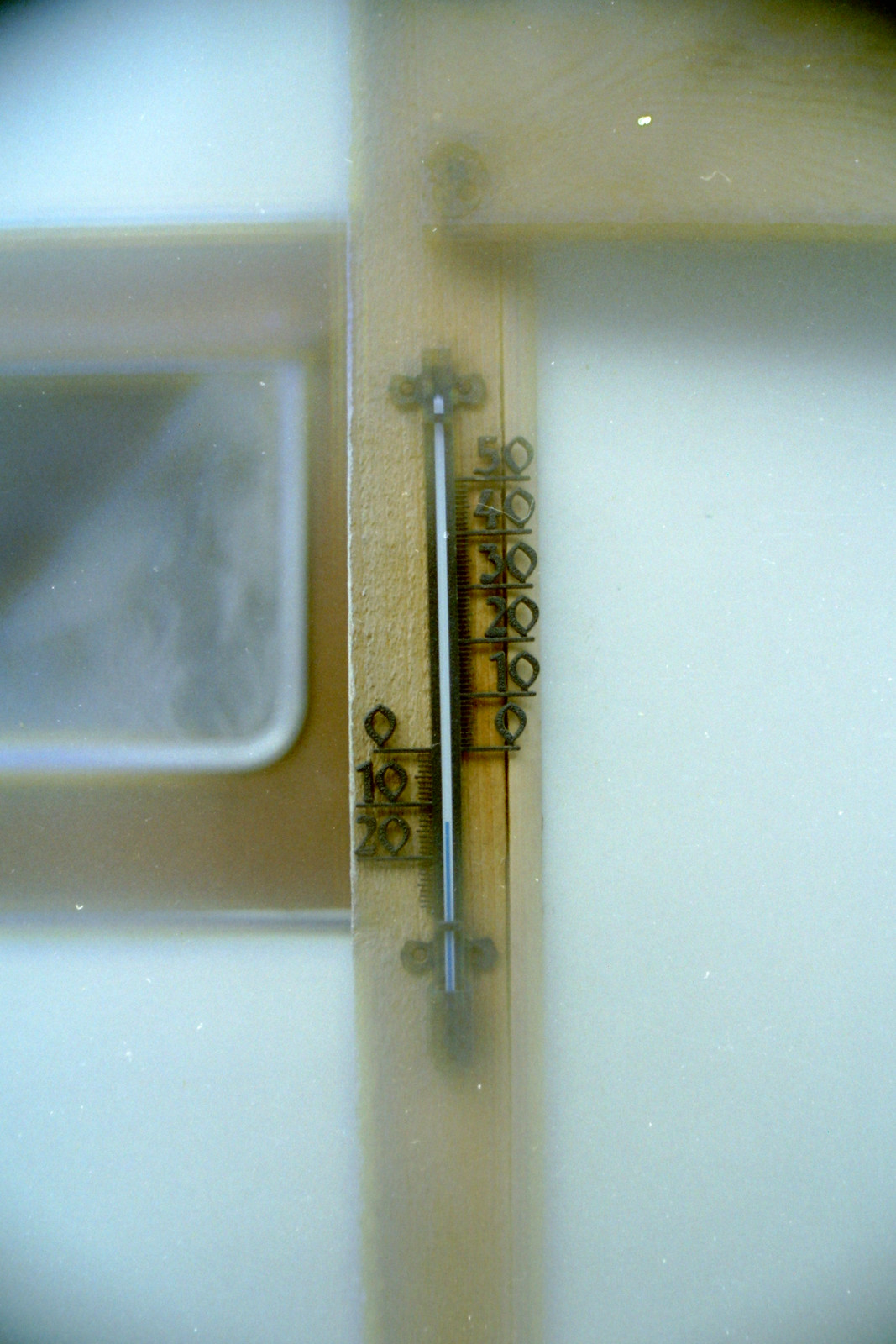The image features a detailed close-up of a black, decorative metal handle affixed to the wooden exterior of a house. The camera is tightly focused on the handle, rendering the background in soft blur. The handle is vertically oriented and divides the image into two halves.

On the right side of the handle, there are six numbers arranged in descending order: 50 at the top, followed by 40, 30, 20, 10, and 0 towards the bottom. On the left side, there are three numbers: 0 at the top, 10 in the middle, and 20 at the bottom. Both sets of numbers are black, matching the handle, and appear to be part of a design that spans the length of this metal feature. The precise and meticulous arrangement of the numbers provides a sense of symmetry and order to the image.